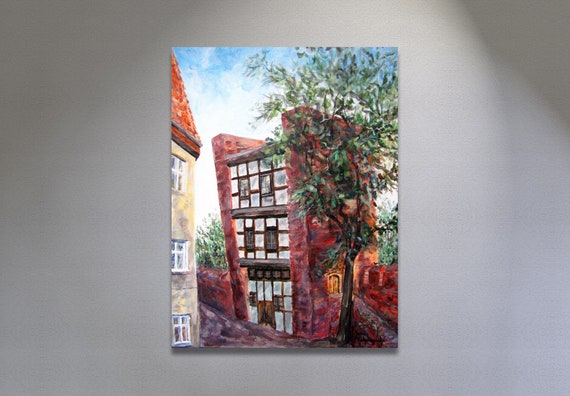The image is a photograph of a painting, which is displayed on a gray wall, possibly within a museum setting. The painting itself, without any frame, is a detailed cityscape focusing on two adjacent buildings under a bright, blue sky with scattered white clouds.

The left portion of the painting depicts the corner of a three-story building constructed from light brown stone and topped with a gabled red roof. The building features white-framed windows on each floor and presents a partial, yet close-up view.

To the right, the primary subject is a three-story building with a distinctive glass facade framed in brown. This structure is flanked by red brick on either side, reinforcing its classic, almost historical appearance. Dominating the right side of the building, a tall tree with a thick brown trunk and abundant green leaves extends above the rooftop, adding a touch of natural elegance to the urban scene.

Additionally, there appears to be a pathway descending alongside the glass-fronted building, adding depth to the composition. The combination of architectural details and natural elements, along with the bright and cloudy sky, frames a dynamic and harmonious depiction of an old cityscape.

This imagery, captured in watercolor style, offers a complex yet coherent blend of urban and natural elements bathed in daylight, presenting a fascinating slice of historical architecture and serene environment.